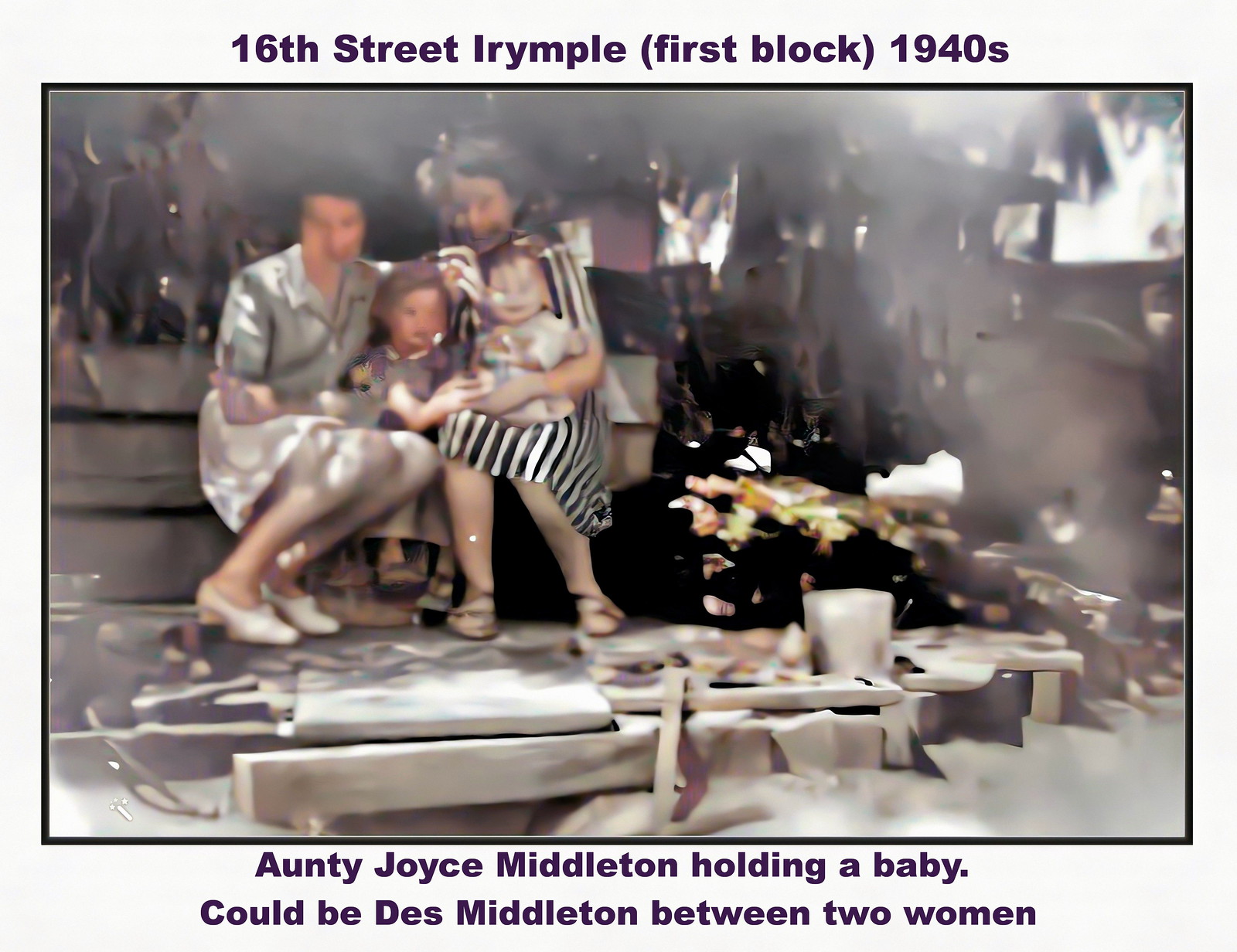This photograph, taken in the 1940s and titled "16th Street Iripole (first block)," captures a poignant family moment on an outdoor staircase, bench, or possibly a partially constructed deck or porch, during the spring or summer. The image features two women, one wearing a plain beige dress and the other in a black and white striped dress, seated closely together with two toddlers. The woman in the striped dress has a baby on her lap. The other toddler sits between the two women. The toddlers, who appear to be around two years old, are dressed similarly; one in a lavender dress with brown hair and the other in a white dress with dark brown hair. The quality of the photograph is quite poor, described as blurry, foggy, and shadowy, with faces hard to discern. An attempt to restore it seems to have been made, but the details remain unclear. In the background, there are trees, a possible porch, and even what appears to be a truck or tractor to the right. The top caption notes the location, and the bottom caption mentions Auntie Joyce Middleton potentially holding one of the toddlers, with a possibility that the baby could be Des Middleton.